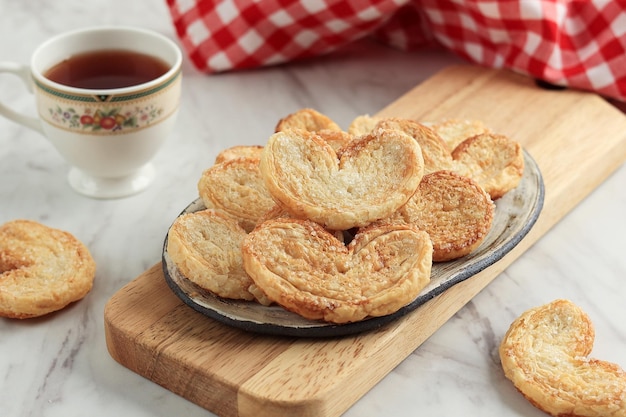The detailed photograph showcases a charming arrangement of heart-shaped cookies and tea. In the center, there are approximately six or seven lightly browned heart-shaped cookies, sprinkled with sugar crystals and displayed on a gray ceramic plate. The plate itself features an intricate greenish-gray floral pattern and a blue rim. This plate rests on a thick wooden cutting board positioned diagonally, creating an inviting presentation.

Surrounding the plate, a few cookies are placed directly on the marble white surface, adding to the scene’s rustic appeal. In the top left corner, a white teacup with green and red floral designs and a green circular band at the rim contains lightly brown tea, complementing the homely setting. In the blurred background, a fragment of a red and white checkered tablecloth is visible, enhancing the cozy, vintage vibe of the setup. The entire scene is well-lit, highlighting the warm, inviting ambiance of the display.